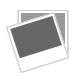This detailed illustration on the cover of a magazine from the 1984 NBA All-Star Game showcases a vibrant, colorized scene of two basketball players mid-jump for the ball. The player on the left, a white man, sports a white jersey with "West All-Stars" emblazoned across it, along with the number 3 prominently displayed. He wears tall white socks with blue stripes and white sneakers with matching blue stripes. The player on the right, a black man, dons a red jersey labeled "East," accompanied by white socks with red stripes and white sneakers featuring blue stripes. Both athletes are depicted against a picturesque backdrop characteristic of Colorado, complete with tall trees, a serene body of water, and snow-capped mountains, echoing the event's host state. The top of the cover reads "1984 NBA All-Star Game" in bold text, with a red star situated between "All" and "Star," and further details are provided near the upper left corner: "McNichols Sports Arena, January 29, 1984." The bottom left corner of the cover notes the price of the magazine: $4 tax included. This artistic rendering, blending elements of sports excitement and natural beauty, is both nostalgic and evocative of the era and event.